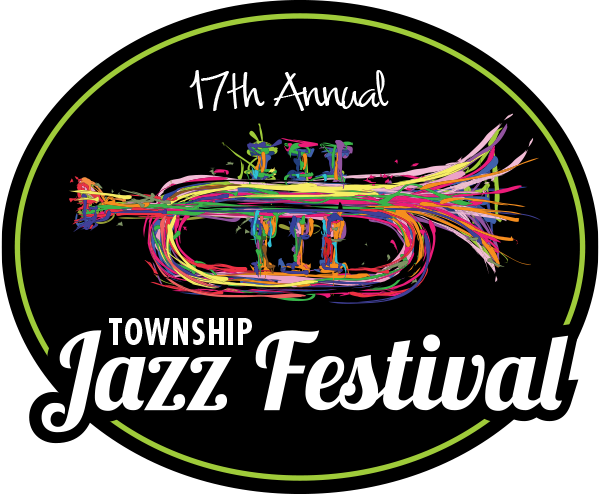The image is an advertisement promoting the 17th Annual Township Jazz Festival. The design is predominantly contained within an oval shape featuring a black background with a green stripe encircling the perimeter. At the top of the graphic, in white font, the text reads "17th Annual." Central to the advertisement is a vibrant, multicolored drawing of a trumpet. The trumpet illustration appears somewhat incomplete, with a mix of yellow, pink, dark blue, green, red, and orange hues, giving it a dynamic, paint-splattered look. This colorful artwork draws significant attention and serves as the focal point. Below the trumpet, in much larger white text, is the event's name: "Township Jazz Festival." Overall, the design has a striking, sticker-like appearance with the bold, rainbow-colored trumpet set against a stark black background accented by the green border.